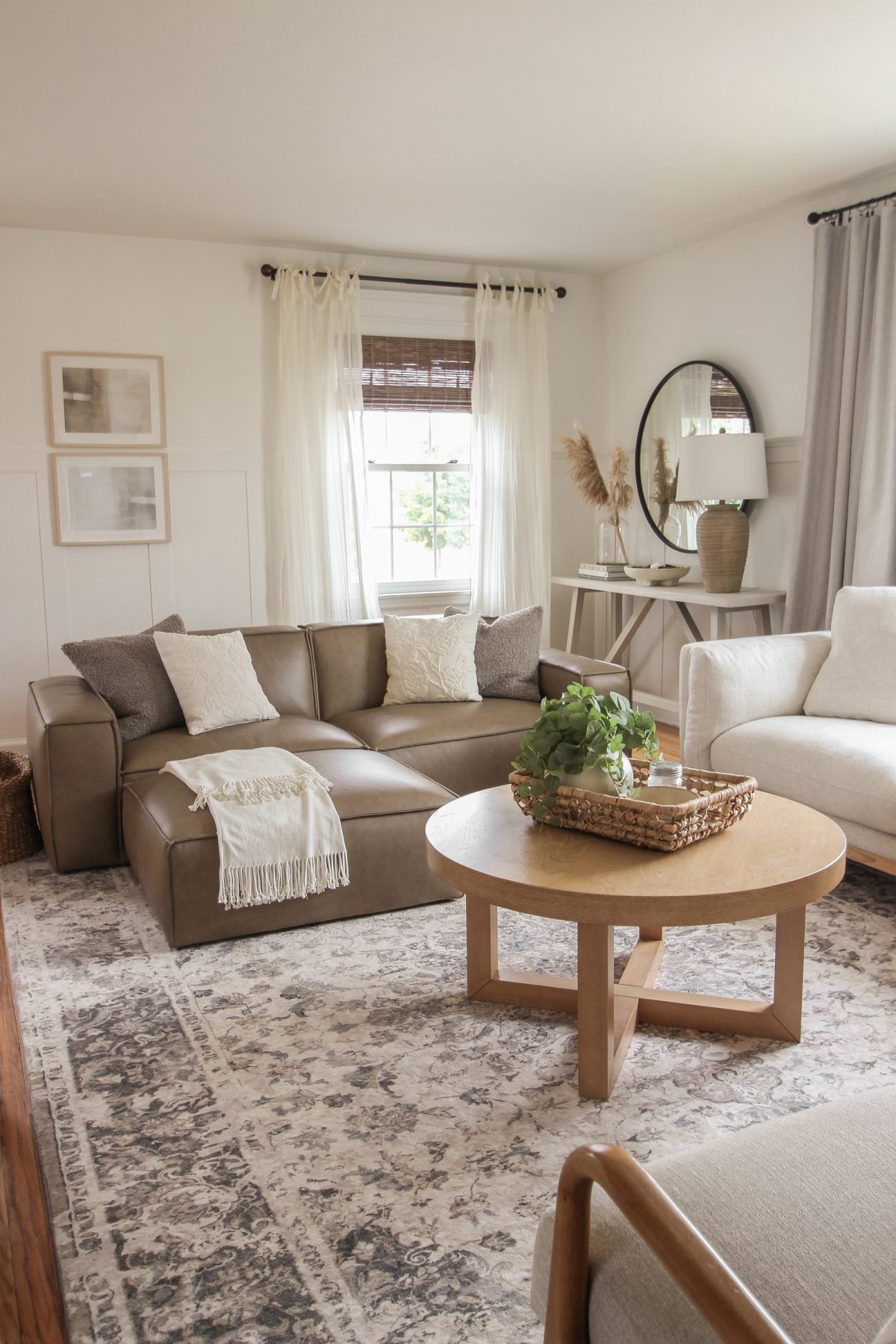This image captures a spacious, country chic living room with elevated white-painted walls and ceilings, likely around nine to ten feet high. The wide wood paneling on the walls and the rich brown hardwood floor create a warm and inviting atmosphere. A room-size wool rug in gray and white floral patterns covers much of the floor, probably measuring around 10 feet by 15 feet.

The seating arrangement includes three distinct sofas: a large brown leather sofa with white and gray pillows and a matching footstool in front of it, a white fabric sofa with tan, cream, and brown throw pillows, and a third white fabric chair with a wooden frame located in the corner. 

In the center of the room, there's a wooden coffee table with unique X-shaped legs and a round top. Atop the table sits a straw basket containing a glass vase with a flower pot and a green plant. Further adding to the charm, there is a table with a brown base and a white lampshade, as well as a circular black-framed mirror mounted on the wall.

The window treatments consist of sheer white curtains behind the leather sofa, complemented by bamboo blinds, all set on black rods. Another picture window, accompanied by grayish curtains on black rods, reveals a view of a bush outside, enhancing the natural aesthetic of the room. The décor is completed with two framed photographs on the wall and various other decorative items, contributing to the room's cohesive brown, white, and gray color palette.